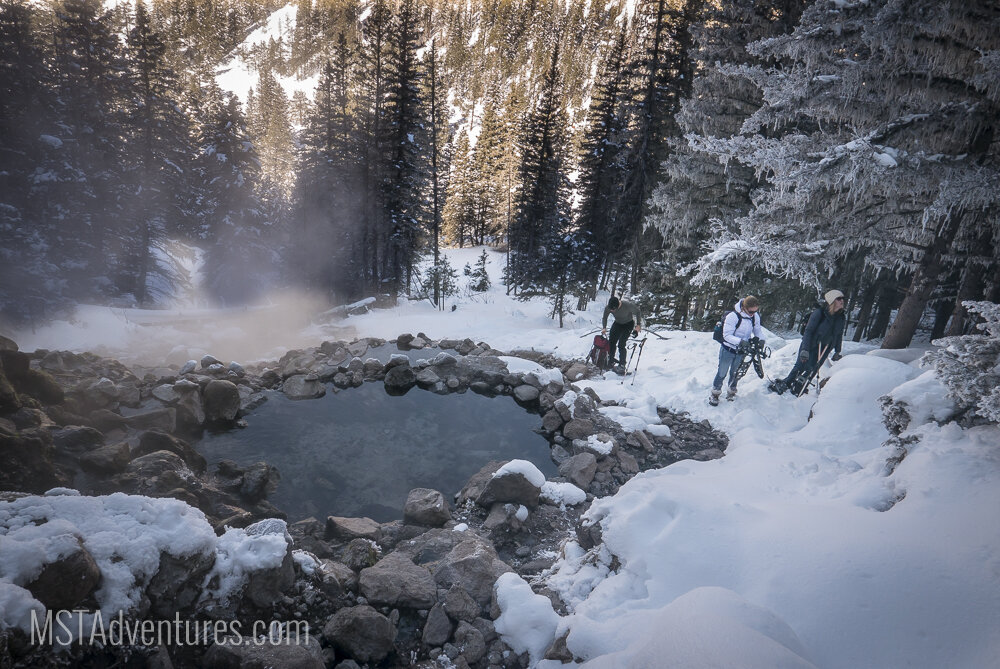The photograph captures a cold, snowy mountain landscape with dense pine trees dotting the hillside. At the center of the image, three adventurers stand out against the white backdrop. Each is equipped with heavy winter gear and skiing equipment. In the foreground, a man in a long-sleeved blue jacket and white beanie stands tall. Beside him, a woman dressed in a white parka, jeans, and boots is notably without a hat. Further in the background, another man, wearing black pants, a thin long-sleeved gray top, and a black cap, is bending over.

To their left, the landscape reveals a curious feature - a steaming hot spring surrounded by bare rocks, conspicuously lacking the snow that covers the rest of the area. The escaping steam hints at the warm temperature of the water amidst the chilly environment. The bottom left of the frame prominently displays the watermark "mstadventures.com," marking the photograph's origin.